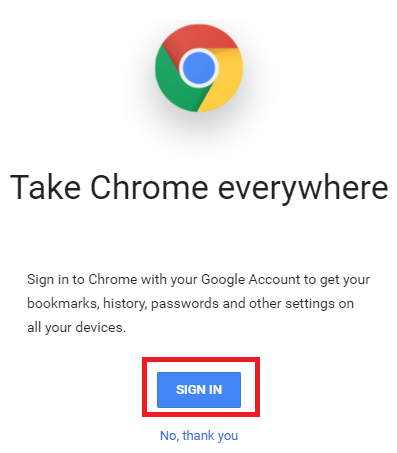The image is a clean, white-background screenshot showcasing a Google Chrome prompt. At the very top, there is the iconic Google Chrome logo featuring a central turquoise blue circle with a white outline. Surrounding this central circle are primary color segments: red at the top, yellow on the right, and green on the left, arranged in a swirling pattern. The logo appears to cast a slight shadow beneath it. Below the logo, in bold font, the text reads "Take Chrome everywhere." Just beneath this, in slightly smaller font, it says, "Sign in to Chrome with your Google account to get your bookmarks, history, passwords, and other settings on all your devices."

Further down, there is a blue rectangular button with the text "Sign in" in white letters, circled by a red rectangle. Below this button, a clickable text option reads, "No, thank you" in blue letters. The entire page maintains a stark white background with no additional elements or edges visible, emphasizing the central content and the Google Chrome branding.